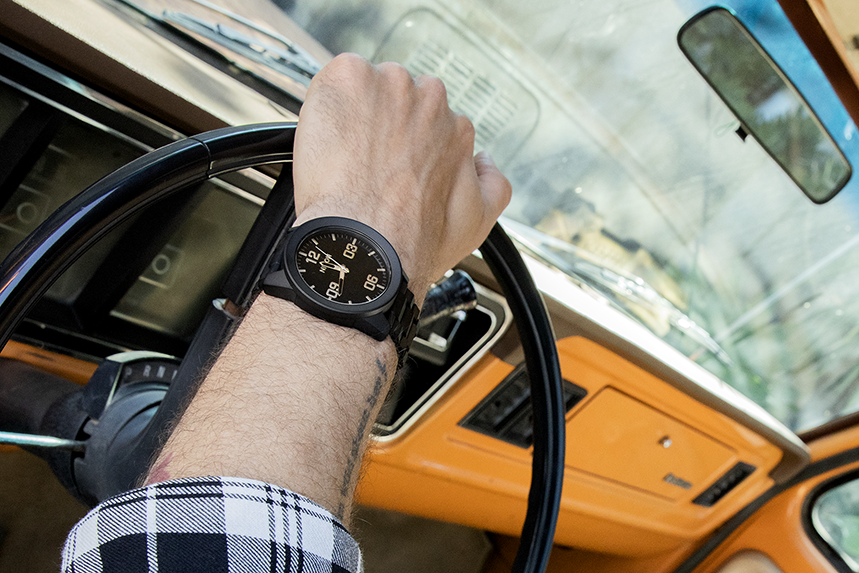The image captures a detailed, close-up view from the driver's perspective inside an older, retro car, possibly from the 70s, resembling a model like the Ford Bronco. The interior is a mix of black and burnt orange, with the dashboard prominently displaying these colors. The windshield is flat, rather than sloped, a characteristic feature of older vehicles. The driver's left hand rests on a thin, black steering wheel, which is positioned on the left side, indicative of an American car. The man, identified by the hair on his arm, wears a striking black and white plaid flannel shirt, revealing a tattoo on his arm. His wrist is adorned with a large, traditional watch that clearly shows the numbers 12, 3, 6, and 9. The gear shifter is intriguingly placed on top of the steering wheel's stem. Although the scene outside the windshield is blurred and indistinct, the focus remains on the car's vintage interior and the driver's arm details. The glove box and part of the dashboard are visible behind the steering wheel, enhancing the retro aesthetic of the car's cabin.